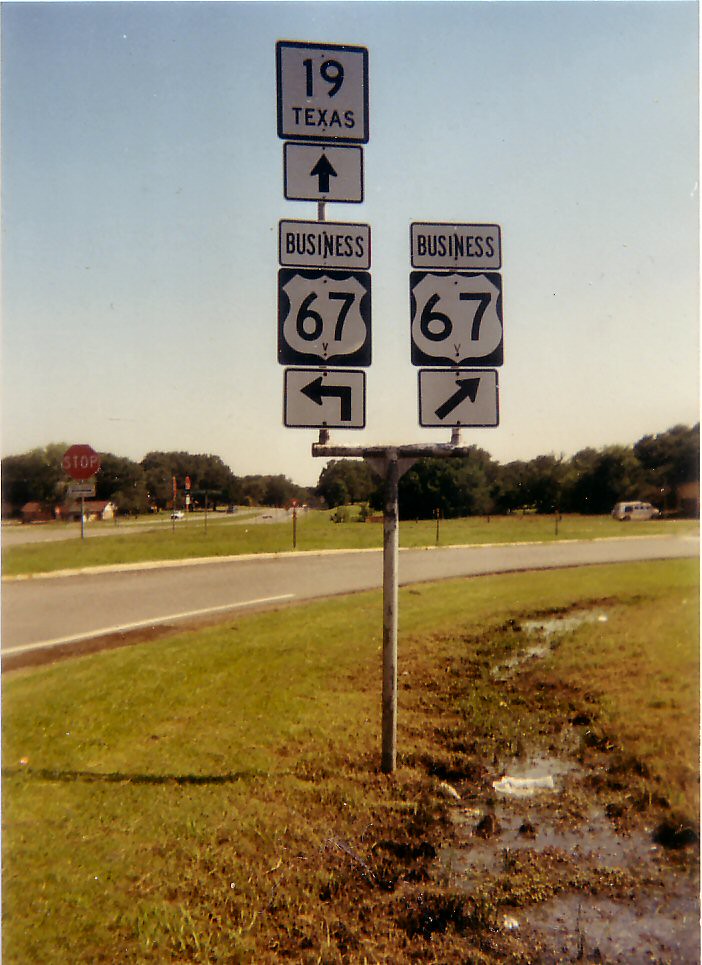The image captures a bright, sunny day in Texas, showcasing a roadway flanked by various highway signs. The scene foreground features green grass with a strip of muddy water running through it, and a grey road patch to the bottom left, curving into the background. Prominently positioned is a grey steel pole supporting multiple highway signs. One sign reads "BUSINESS" with a black-lined shield displaying "67" and a black arrow pointing to the right. Adjacent to it, another sign features "19 Texas" with an upward arrow and "BUSINESS 67" with a left-pointing arrow beneath it. In the background, left of the signs, stands a small stop sign and a patch of trees, with a blue sky overhead. Further back, a bus and more trees are visible, along with a distant highway and a small house, capturing the tranquil yet structured layout of this Texan scene.